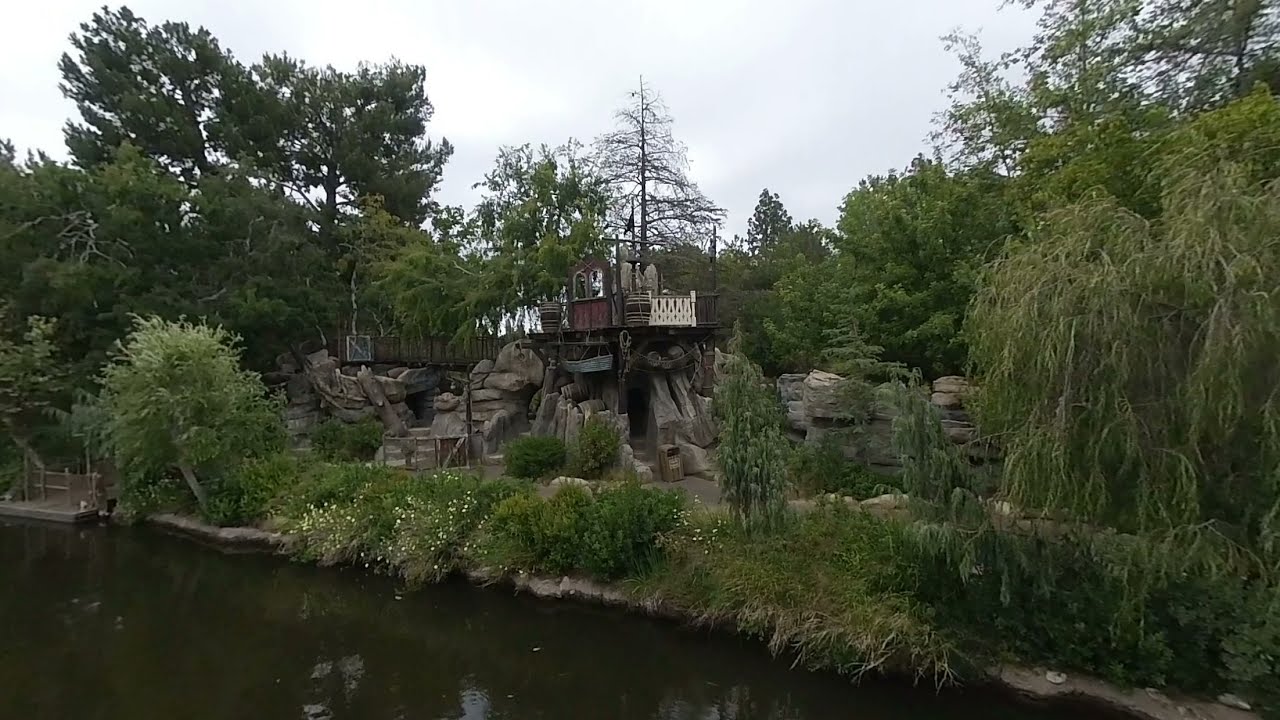In this picturesque outdoor scene, lush greenery abounds, indicating a springtime, summer, or early fall setting. The vibrant foliage, in full bloom, frames a central man-made structure comprised of large rocks and boulders carefully stacked and integrated into the natural landscape. Rising from the stone foundation is a wooden platform adorned with white fencing, resembling elements of a minigolf course, especially with its whimsical and inviting design.

The platform features small windows and an open-air setting, with no visible roof, suggesting it is a vantage point or an area for leisurely exploration. A smooth walking surface surrounds the structure, providing ample space for visitors to meander and take in the scenic surroundings.

At the edge of the greenery, a body of water, possibly a lake or pond, reflects a dark and murky green hue. In the foreground, this water body seems to host a quaint little dock to the far left. The clear sky above, streaked with wispy clouds, completes the serene and idyllic atmosphere of the landscape, blending human craftsmanship seamlessly with nature's beauty.